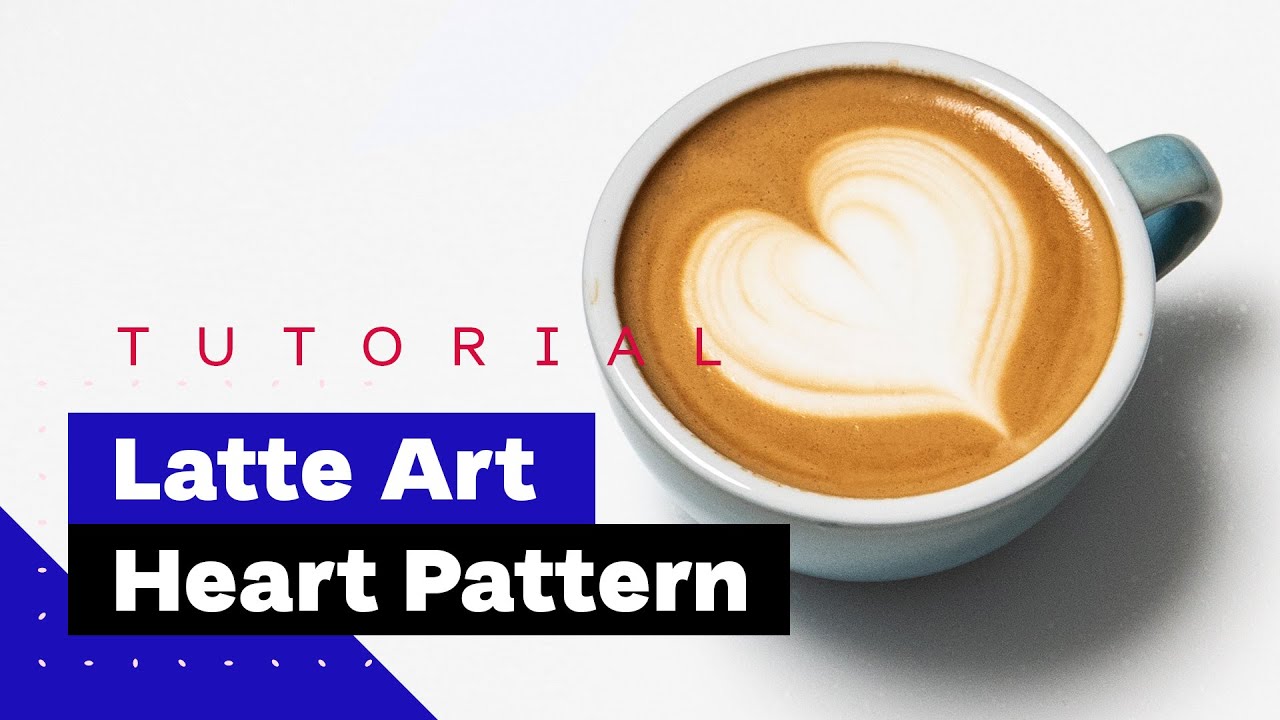The image appears to be a cover for a tutorial video, featuring a detailed photograph taken from above of a ceramic coffee mug. The mug contains brown coffee with a white heart shape intricately created with milk on its surface. The coffee mug is grey with a handle that has a bluish tint, set on a clean white background, casting a subtle shadow to the bottom left. On the top left corner of the image, the word "Tutorial" is prominently displayed in red text. Below it, "Latte Art" is written in white on a thick blue banner, and beneath that, "Heart Pattern" is inscribed in white on a black banner. Additionally, the bottom left corner of the image features a blue section adorned with a pattern of white dots arranged in a grid.